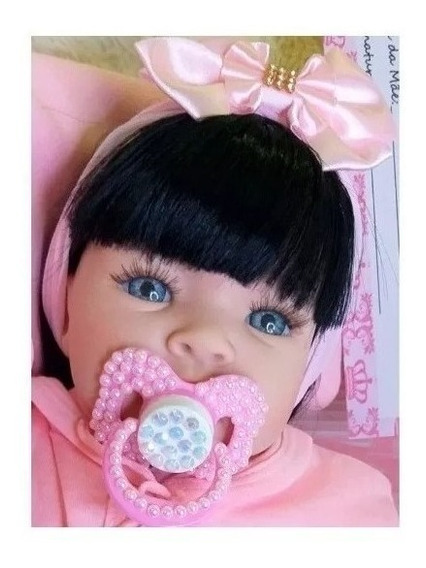This image depicts a lifelike baby doll with detailed features. The doll has dark black hair, long black eyelashes, and striking blue eyes. It has a pug nose and holds a pink pacifier in its mouth. The pacifier is adorned with medium pink pearls and a white center with silvery sequins. The doll is accessorized with a pink ribbon or bow that wraps around its head, covering even its ears. Dressed in a pink outfit, possibly a hoodie or onesie, the doll is lying face up on a pink pillow. The setting appears to be indoors on a cream-colored carpet. Behind the doll, there is what looks like a gift card or form, decorated with pink crown logos. The colors in the scene include shades of pink, white, gold, light blue, black, gray, and light pink.